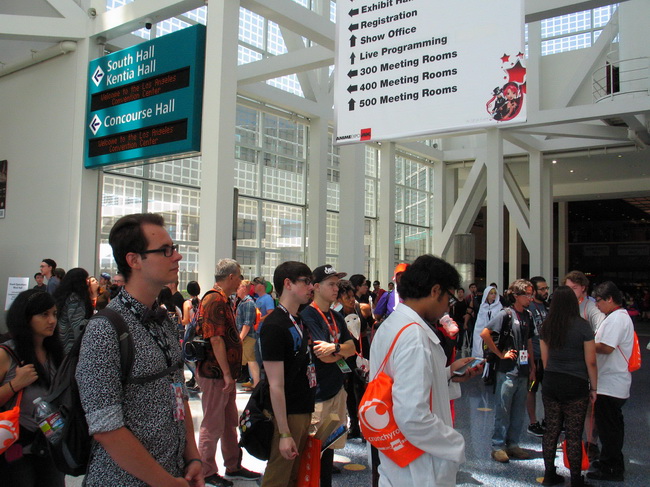The image depicts a bustling convention center filled with numerous attendees, many of whom are sporting distinctive Crunchyroll bags, indicating an anime convention. The convention center’s interior is characterized by its numerous white columns, off-white walls, and extensive glass windows that offer a view outside, suggesting it is daytime. Dominating the scene is a large sign on the right side with directional arrows pointing towards various locations, including "Exhibit", "Registration", "Show Office", "Live Programming", "300 Meeting Rooms", "400 Meeting Rooms", and "500 Meeting Rooms". Another sign on the left mentions "South Hall", "Kenta Hall", and "Concourse Hall", with arrows guiding attendees. The crowd, mostly facing right, includes notable individuals such as a man with a black and white shirt carrying a black backpack with a water bottle, a man wearing glasses and tan pants, a person in a navy blue shirt with an orange pocket holder around his neck, and another in a white coat with a Crunchyroll logo. The scene captures the vibrant, crowded atmosphere of the convention, with people scattered all throughout the entryway.